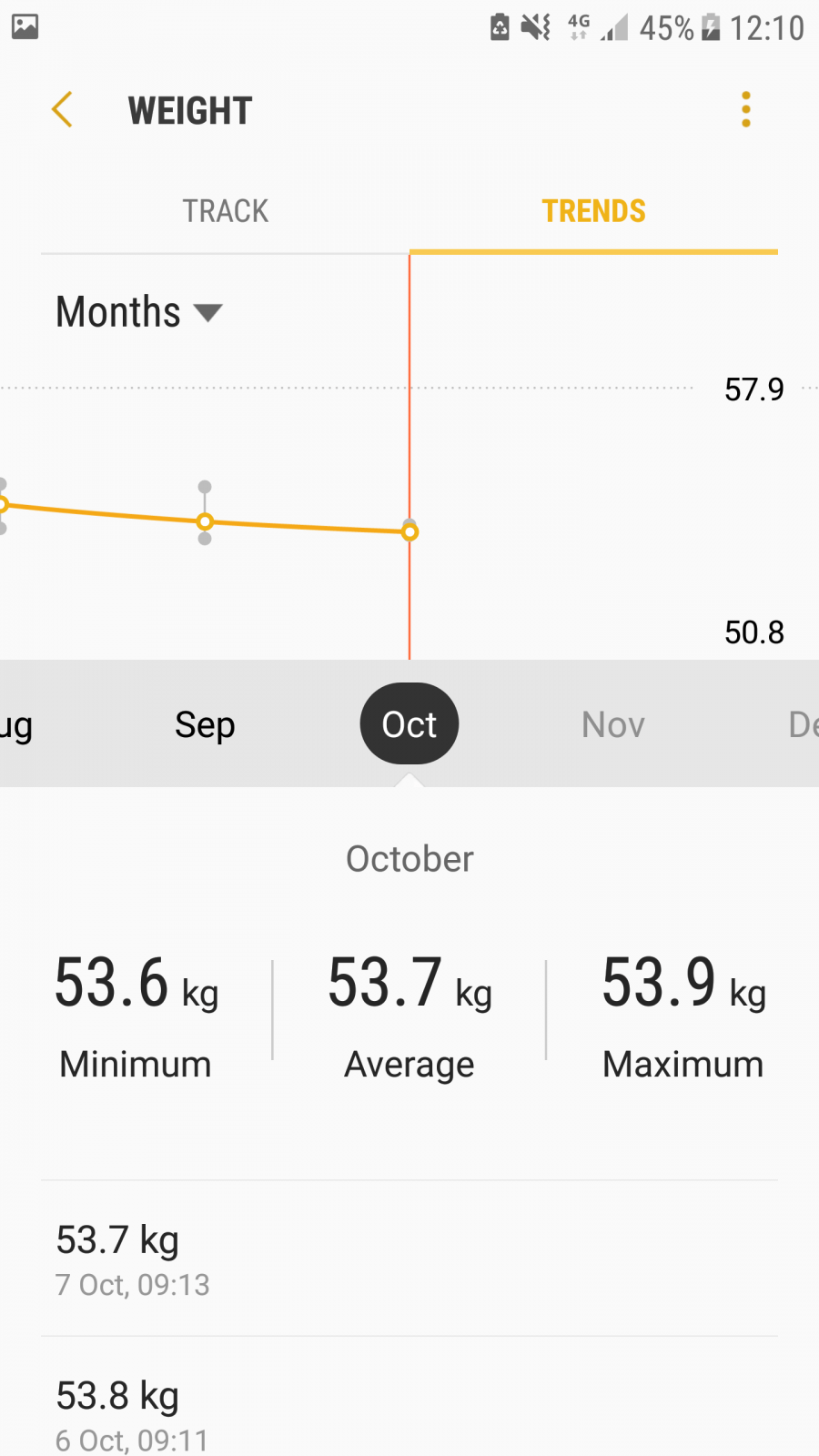The image shows a smartphone screen displaying a package tracking and weight trend analysis interface. At the top of the screen, the word "Wait" is prominently displayed in black, with an accompanying orange arrow. Below this, there are two buttons: "Track" and "Trend." The "Trend" button is highlighted in orange, indicating it is the active selection.

The main part of the screen features a line graph that tracks weight changes over several months: August, September, October, November, and December. Currently, the focus is on October. The graph begins in August with an orange line, which seems to dip as it moves into September. From September to October, a red trend line sharply rises and then levels off, showing a significant weight change.

Above and below the trend line in October, numerical data points are labeled. The top mark indicates 57.9, and the bottom mark indicates 50.8. The word "October" is prominently highlighted in black in the middle of the graph area, with the text in gray.

Additional data is presented below the graph, denoting minimum, average, and maximum weights for the period. The minimum weight recorded is 53.6 kg, the average is 53.7 kg, and the maximum is 53.9 kg. Specific dates and times are also listed: 53.7 kg on October 7th at 9:13 AM and 53.8 kg on October 6th at 9:11 AM.